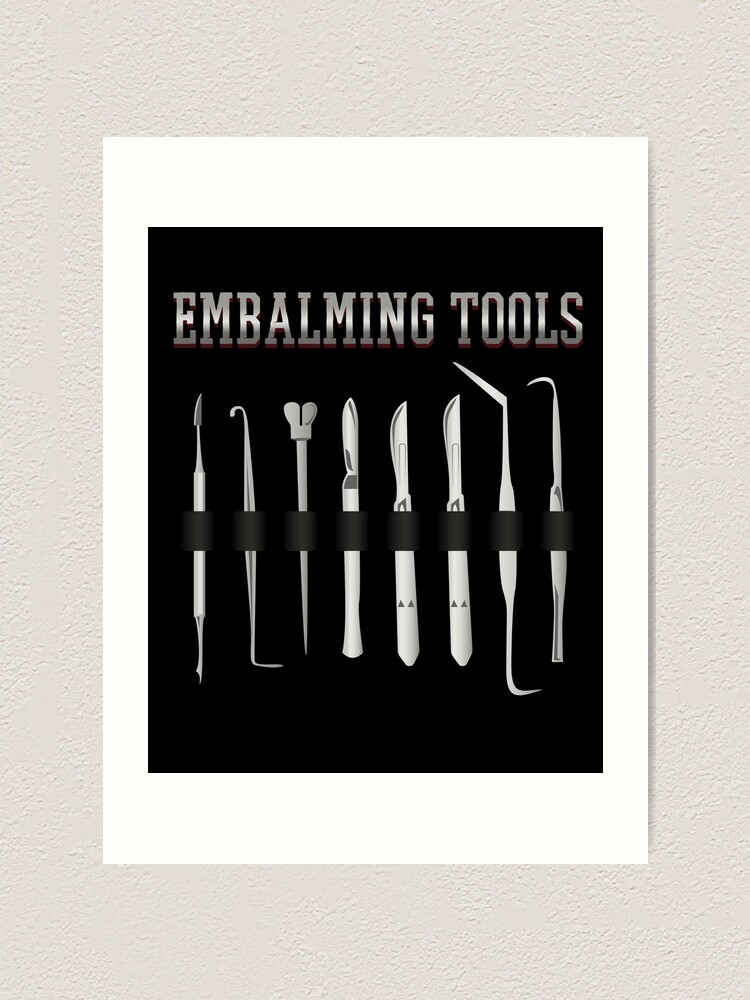This detailed color photograph captures a poster displaying various embalming tools. The poster hangs on a tan, cream-colored wall with a distinctive popcorn-textured ceiling border above it. The white rectangular frame of the poster contains a solid black rectangle inside, which vividly contrasts the surrounding. At the top of the black rectangle, the title "EMBALMING TOOLS" is prominently displayed in large silver letters. The centerpiece of the poster features eight different embalming instruments arranged from left to right. The tools, all rendered in a silver-gray color, include a variety of scalpels, a pick, a cuticle pusher, and a shepherd's hook-like tool. Despite their distinct shapes and sharp metallic edges, none of the tools are individually labeled.